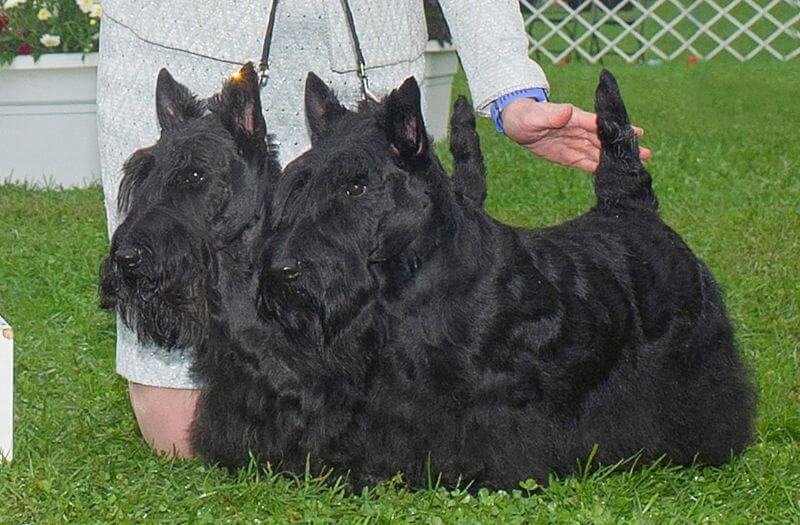In the photograph, two entirely black Scottish Terriers, their long fur cascading down to the ground, stand attentively on a lush green grass tuft. Their tails are perked up, pointing towards the sky, as if they are in a show presentation. Positioned behind them is a woman, presumably their owner or handler. She is dressed in a coordinated dress and shirt combo, with the skirt reaching down to her thighs. Her left hand gently touches the tails of one of the dogs, while her right hand is obscured from view, but you can see two leashes extending from the dogs' necks up towards her. The dense fur of the terriers hides their legs entirely. In the background, there is a distinct gray, thatched fence and a few flowers can be seen growing off to one side, adding a touch of color to the scene. The image captures a moment of poised elegance and attentive training.